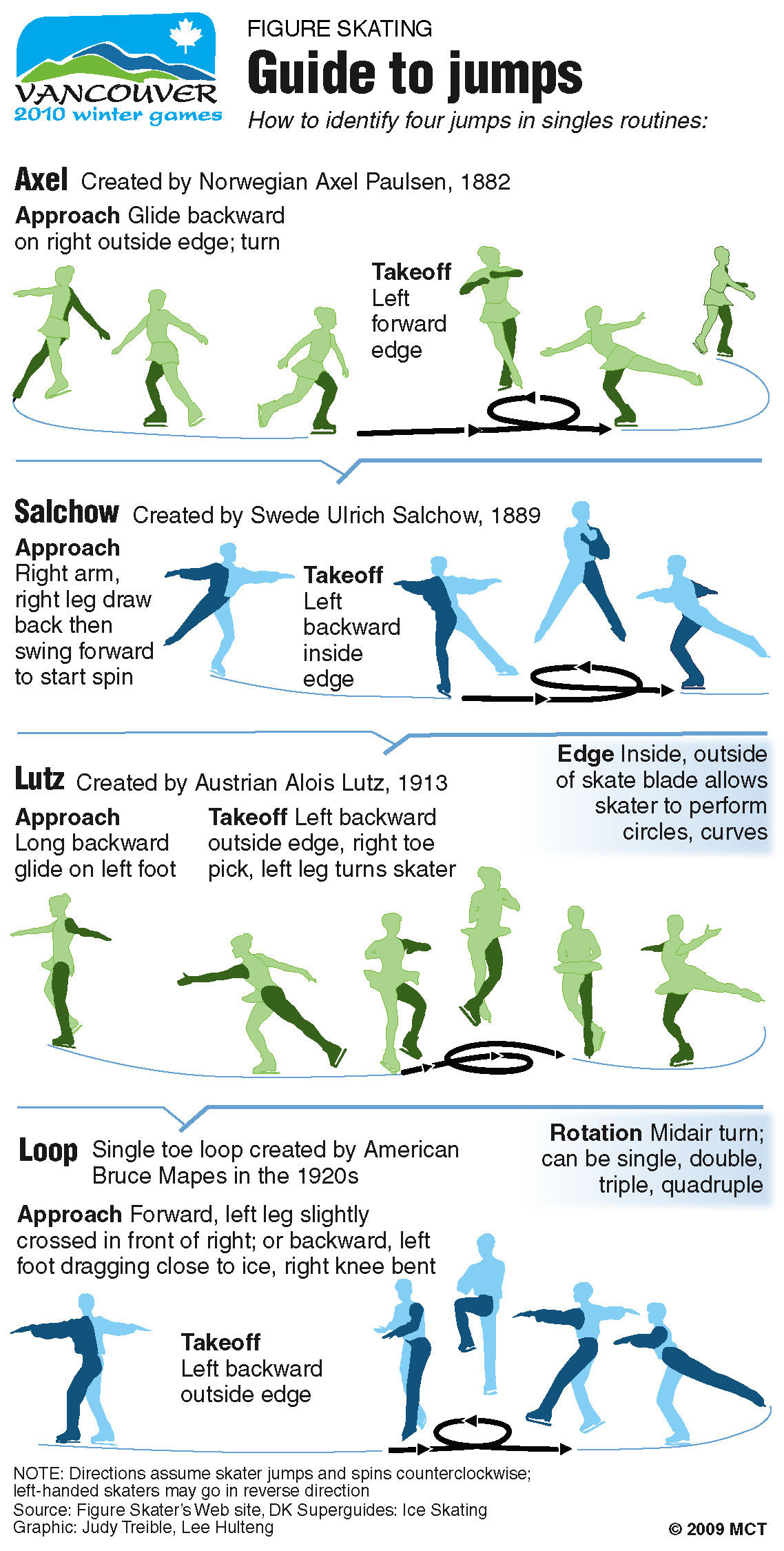This 2009 copyright image from MCT, which resembles a pamphlet or poster, serves as a detailed "Guide to Jumps" in figure skating. Titled "Figure Skating: How to Identify Four Jumps in Single Routines," it was created for the Vancouver 2010 Winter Games. The top section features text in black that introduces the guide and the four jumps: Axel, Salchow, Lutz, and Loop. Each section includes detailed descriptions along with schematic diagrams depicting the execution of each jump by sketched figures, which are colored green for women and blue for men.

- The **Axel**, created by Norwegian Axel Paulsen in 1882, shows the skater gliding backwards on the right outside edge, turning, and taking off from the left forward edge.
- The **Salchow**, originating from Swedish Salchow in 1889, depicts the skater starting with the right arm and leg drawn back, then swinging forward to initiate the spin, and taking off from the left backwards inside edge.
- The **Lutz**, invented by Lux in 1913, illustrates a longer backward glide on the left foot, a takeoff from the left backwards outside edge with the right toe pick, allowing the skater to perform curves and circles.
- Finally, the **Loop**, a single toe loop created by American Bruce Mapes in the 1920s, presents the movement and iconic edge technique used in this jump.

The visual and textual instructions combine to offer a comprehensive guide for identifying and understanding these fundamental figure skating jumps.